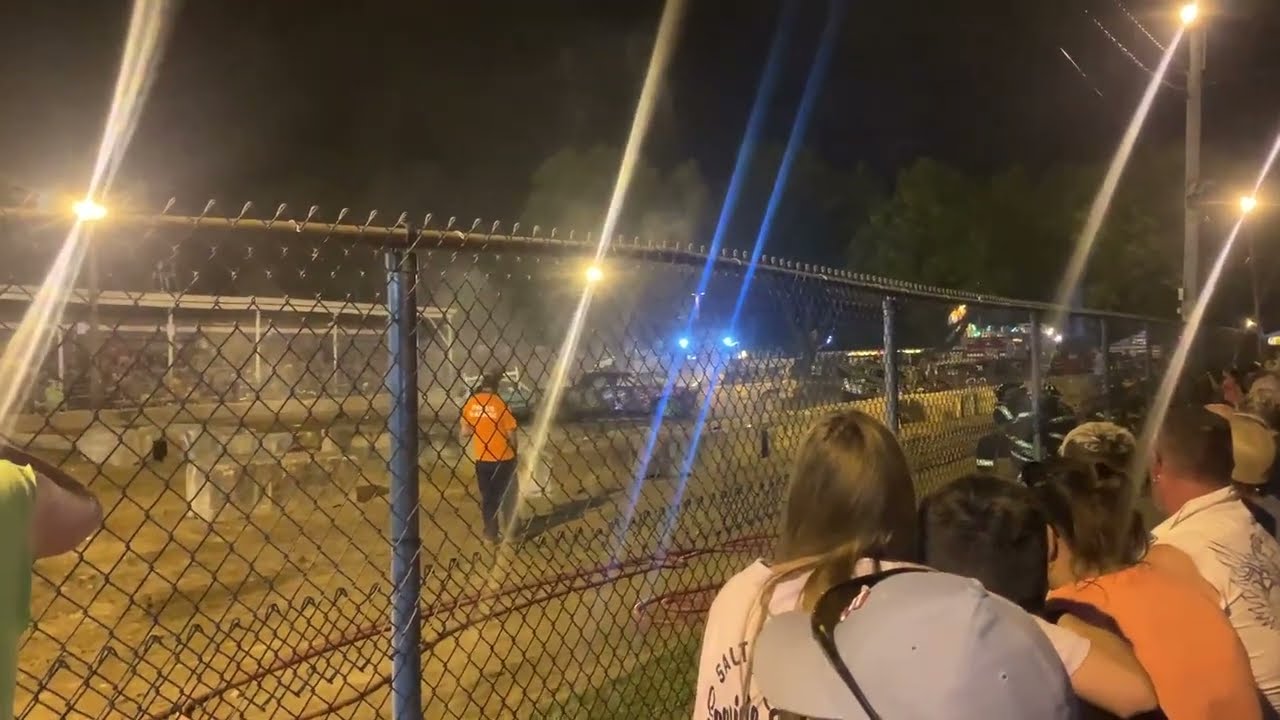This photograph captures a nighttime sports event at a park, set against a black night sky illuminated by streaks of white and blue light. In the foreground, a group of spectators is seated near a chain-link fence, intently watching the activity on the field. This group includes a woman with brown hair, a man in a black shirt, a person with a gray cap, a woman possibly in an orange shirt, and a man in a white shirt. Positioned prominently in the center of the image, behind the fence, is a man dressed in an orange shirt and black pants, which could indicate he is part of the event's staff. The background reveals stadium lights that cast a glow on the field, a building, and distant trees. While specifics of the game or event are unclear, the setting evokes a vibrant yet mysterious atmosphere typical of nighttime park activities.